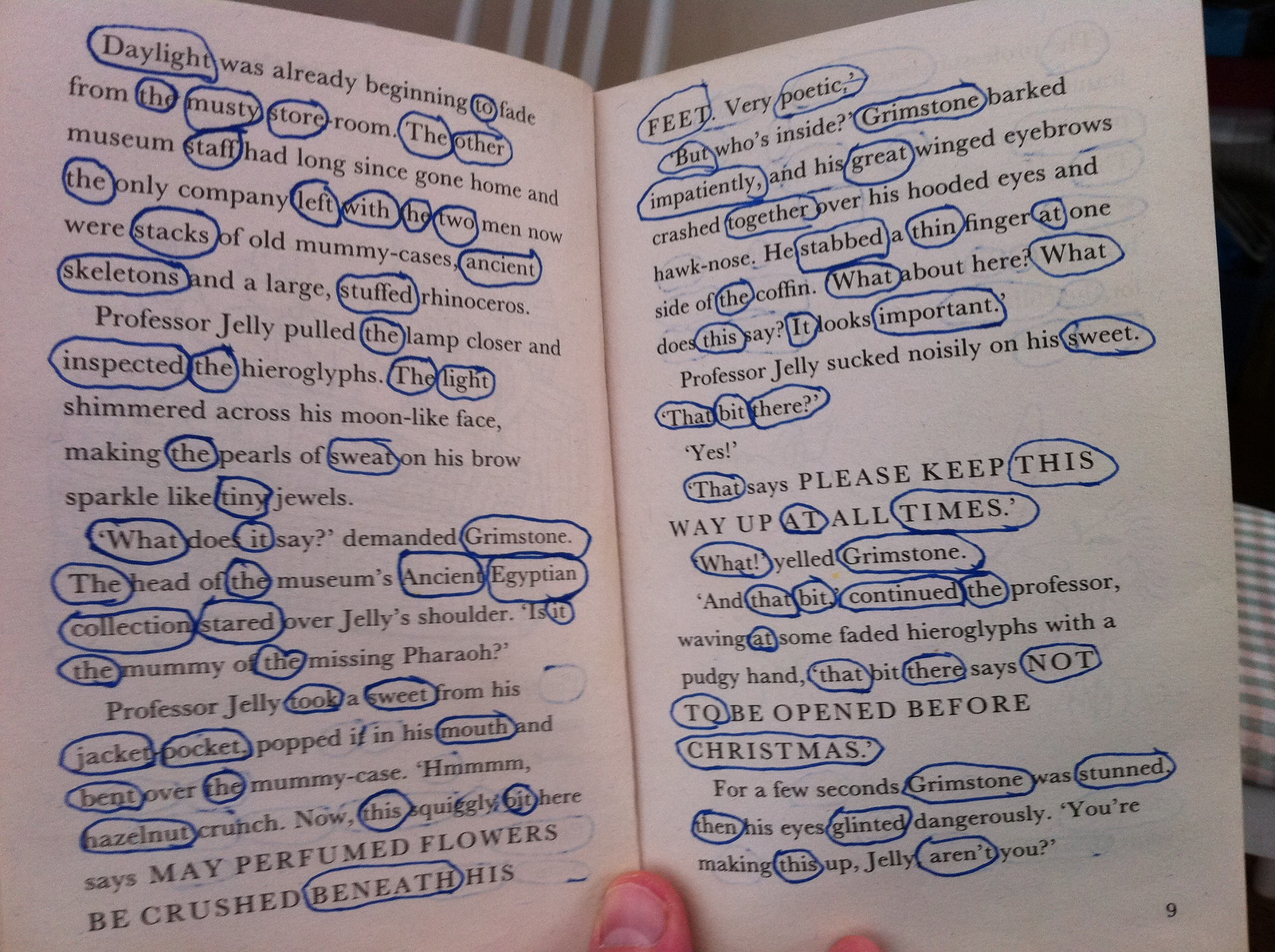The image depicts a close-up of a person holding open a small paperback book, with their fingers visible at the bottom. The book's interior is a stark white background filled with black text. Many words, approximately a third to a quarter of those visible on the two pages, have been circled in blue pen. The visible text on the left-hand page begins with, "Daylight was already beginning to fade from the musty storeroom. The other museum staff had long since gone home, and the only company left with the two men now were stacks of old mummy cases, ancient skeletons, and a large stuffed rhino." The passage continues, detailing Professor Jelly's inspection of hieroglyphs and his interaction with Grimstone, head of the museum's ancient Egyptian collection. The right-hand page contains additional text, and at its bottom, the page number nine is visible. The meticulous circling of words throughout adds a layer of mystery to the scene.